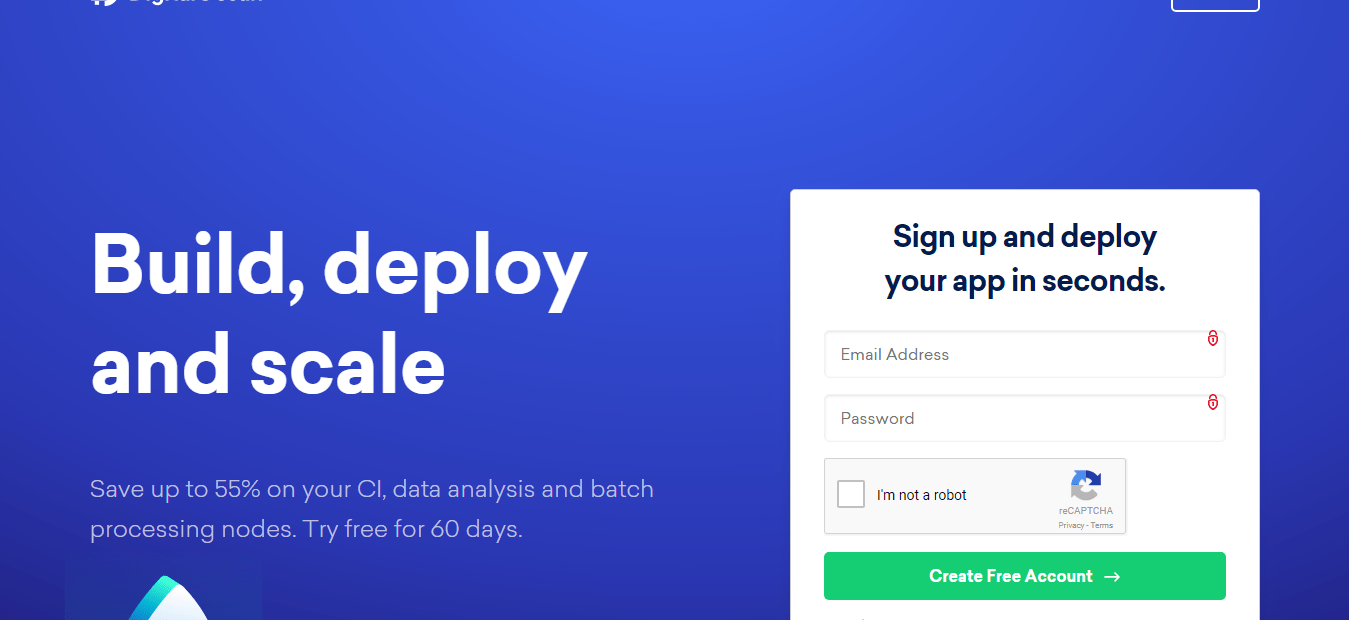The image displays a blue-themed signup page for a website, primarily featuring promotional content and a registration form. On the left side, a bold white text states, "Build, Deploy, and Scale," followed by a promotional offer: "Save up to 55% on your CI data analysis and batch processing nodes. Try free for 60 days." The right side of the image showcases a prominent signup form contained within a white box. At the top of the form, in black font, it reads, "Sign up and deploy your app in seconds." Below this header are fields for entering an email address and password. Beneath the password field, a gray captcha box labeled "I'm not a robot" is present, requiring users to complete a puzzle or test to proceed. At the bottom of the form, a green button with white text and a right-pointing arrow invites users to "Create Free Account."